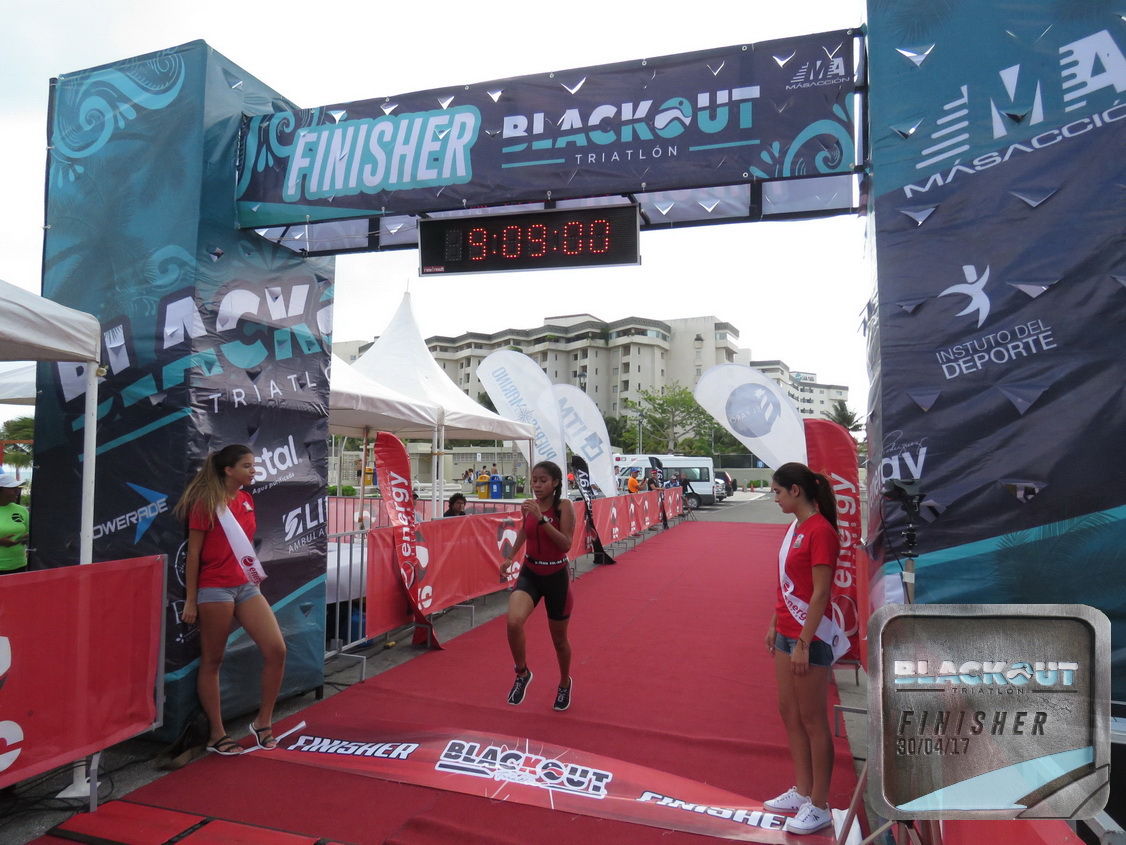The photograph captures the dramatic climax of a triathlon at the precise moment a girl crosses the finish line. Central to the image is the girl, clad in a t-shirt and black shorts, running confidently beneath an imposing blue arch adorned with multiple logos and white highlights. The arch prominently displays the text "Blackout Triathlon" and "Finish," alongside the name "Institute to Del Deporte." Suspended from the arch above her is a digital timer showing 9:09:00. Flanking her are two young girls, each dressed in a red t-shirt, blue shorts, and sporting a white sash over their shoulders, standing attentively near the finish line. A vibrant red mat extends to the finish, bordered by a red fence on the left, with white tents partially visible near the boundary. In the background, a large grey building looms, providing a stark contrast to the vividly colored elements in the foreground. Additionally, a grey rectangle near the bottom right corner bears the logo "Blackout Triathlon Finisher 30.04.17," further emphasizing the event's branding.